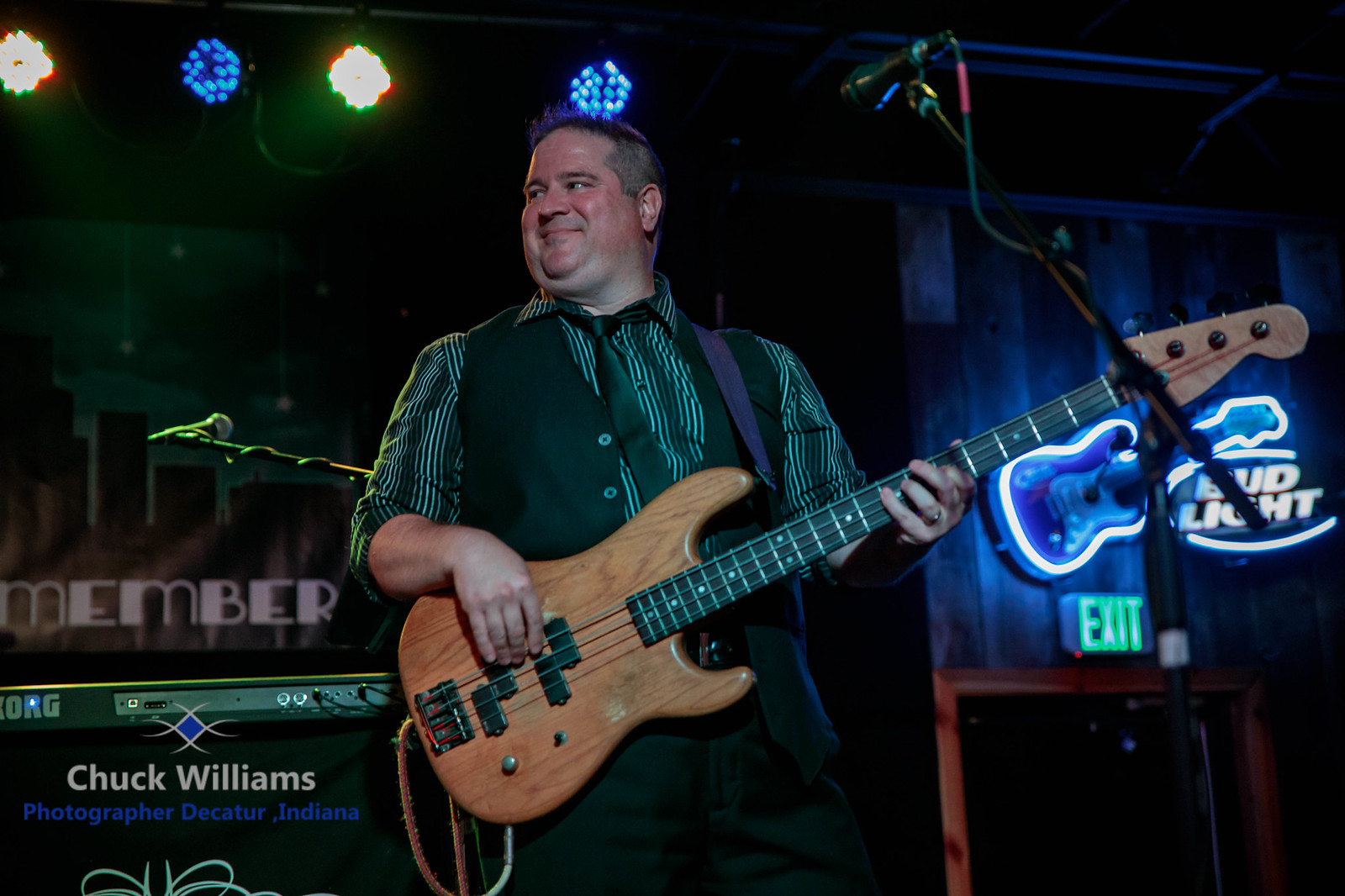In this image taken by Chuck Williams, a photographer from Decatur, Indiana, we see a white male bass player performing on stage, likely in a nightclub or bar setting. He is dressed in a stylish green and black striped long-sleeve shirt with the sleeves rolled up, a black vest adorned with green buttons, a black tie, and black pants. He has short hair and is smirking slightly as he looks to his right, with a microphone positioned in front of him. 

The bass guitar he is playing is a natural wood grain four-string bass with visible pickups and a simple design, featuring only a volume knob and one switch. Behind him, there are various stage lights—yellow, blue, green, and white—that create a vibrant atmosphere. In the background, a Bud Light neon logo and a lit-up guitar sign can be seen alongside a green exit sign above a door. Additionally, there is a keyboard setup behind him, adding to the stage arrangement. The lower left corner of the image bears the watermark: "Chuck Williams, photographer, Decatur, Indiana."